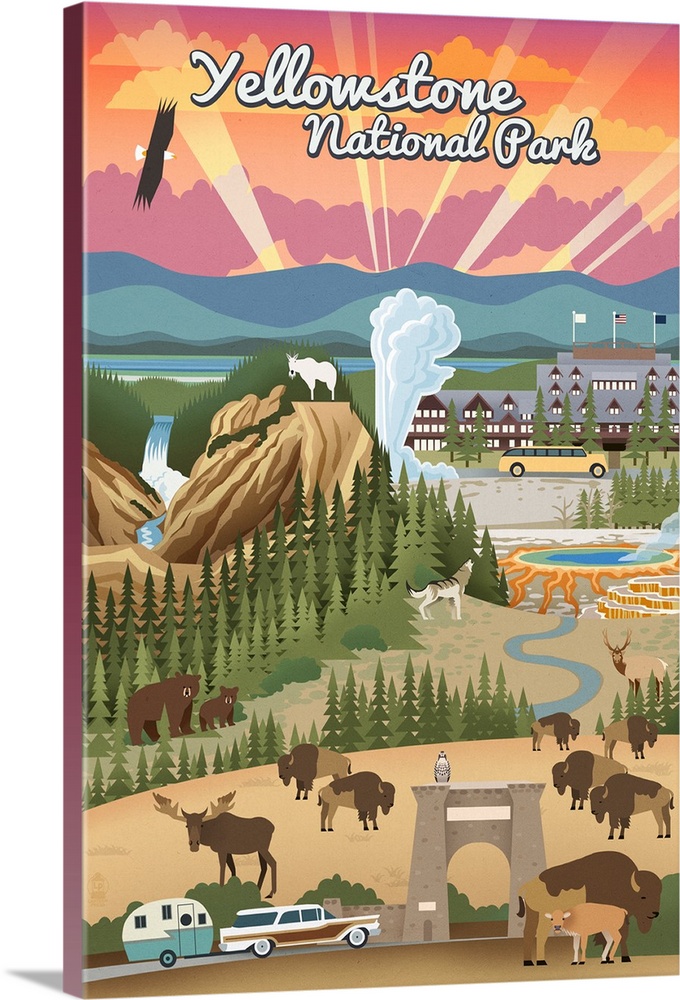This animated image, likely digitally created, appears to be a panel for a Yellowstone National Park booklet or magazine. The scene is a detailed, vibrant landscape setting, angled slightly for effect. At the top, “Yellowstone National Park” is written in elegant white cursive text over a sky filled with shades of pink, orange, and purple, with dramatic sun rays piercing through.

Beneath the colorful sky, dark blue mountain ranges create a majestic backdrop to a thin, reflective lake. Jagged greenery representing mountaintops and hills surrounds a prominent gray building resembling a main lodge. Nearby, there is a noticeable white animal perched on greenery. Flowing through the rugged terrain is a small river, adding a dynamic sense of movement to the landscape.

The scene is rich with wildlife: bears, moose, deer, bison, wolves, and even an eagle soaring in the sky. A distinctive feature is a smoking geyser or volcanic area with fiery red elements, contrasted by a yellow bus stationed to the right of the building. In the lower right corner, a bright yellow bus stands out, while the lower left corner includes a nostalgic wood-paneled station wagon towing a small trailer. The bottom part of the image also depicts a forest backdrop with an archway and various trees, creating a complete, animated representation of what visitors might expect to see in Yellowstone National Park.